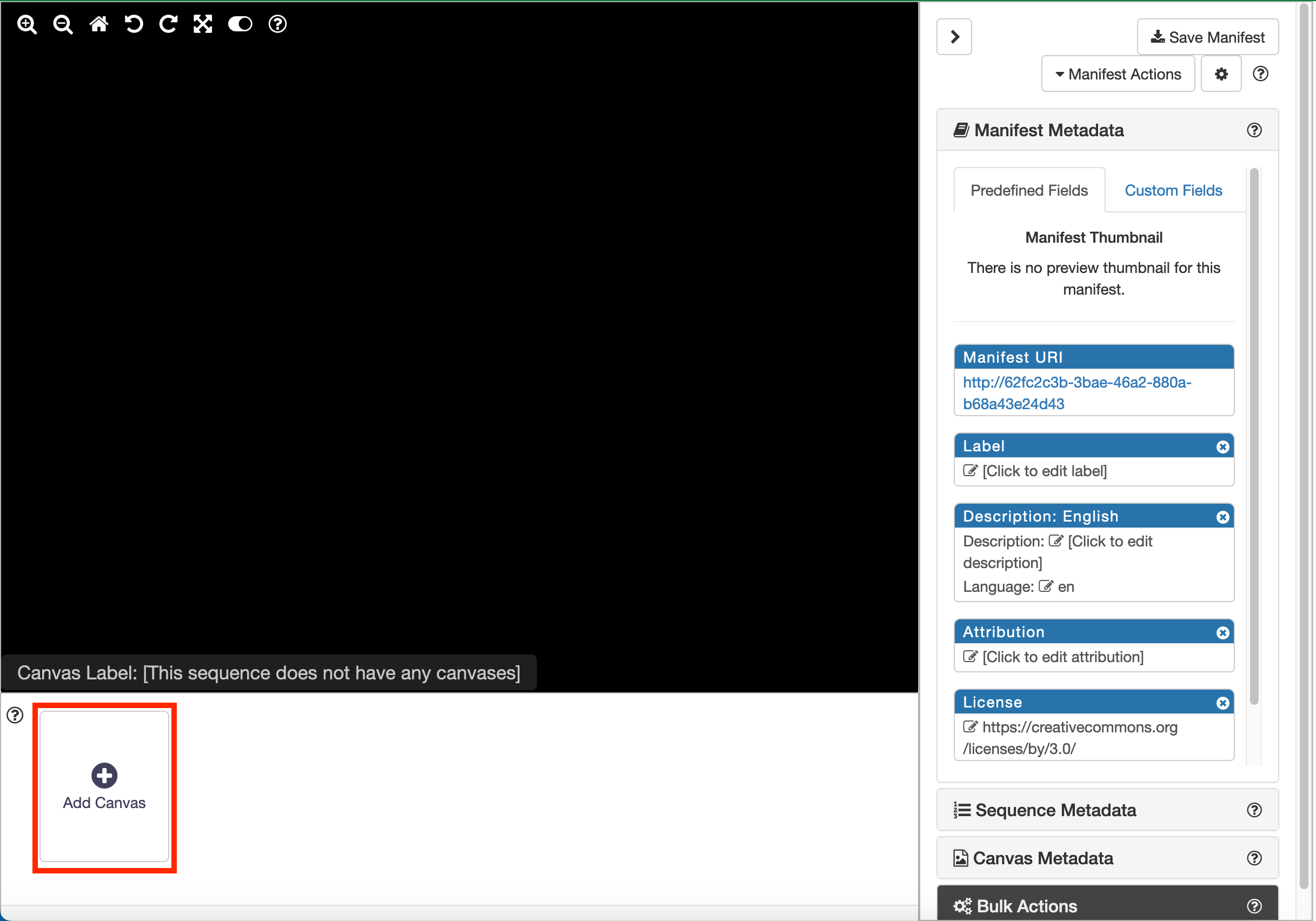The interface displays a variety of icons and text elements with specific functions:

**Top Left:**
1. **Icons:**
   - Plus magnifying glass
   - Minus magnifying glass
   - Building
   - Left rotation
   - Right rotation
   - X (likely to close the element or window)
   - Full screen toggle

**Center:**
- A large black square dominates the center of the interface.

**Bottom Left:**
- A gray rectangle labeled "canvas label" with a message in brackets stating "this sequence doesn't have any canvases"
- Red-bordered area with the label "add canvas"

**Top Right:**
1. **Buttons/Links:**
   - "Write"
   - "Save manifest"

2. **Sections:**
   - "Manifest actions"
   - "Manifest metadata"
     - **Fields:**
       - Predefined fields
       - Custom fields
     - **Thumbnail:**
       - "Manifest thumbnail" with a note indicating "no preview thumbnail for this manifest"
     - **Details:**
       - "Manifest URI," "label," "description" (with a language option and editable description in English)
       - "Attribution," "license" [(https://creatorcommons.org/licenses/by/3.0)]

**Bottom Right:**
1. **Metadata Sections:**
   - "Sequence metadata"
   - "Canvas metadata"
   - "Bulk actions"
   
2. **Icons:**
   - Circle with a question mark

**Background:**
- Predominantly white.